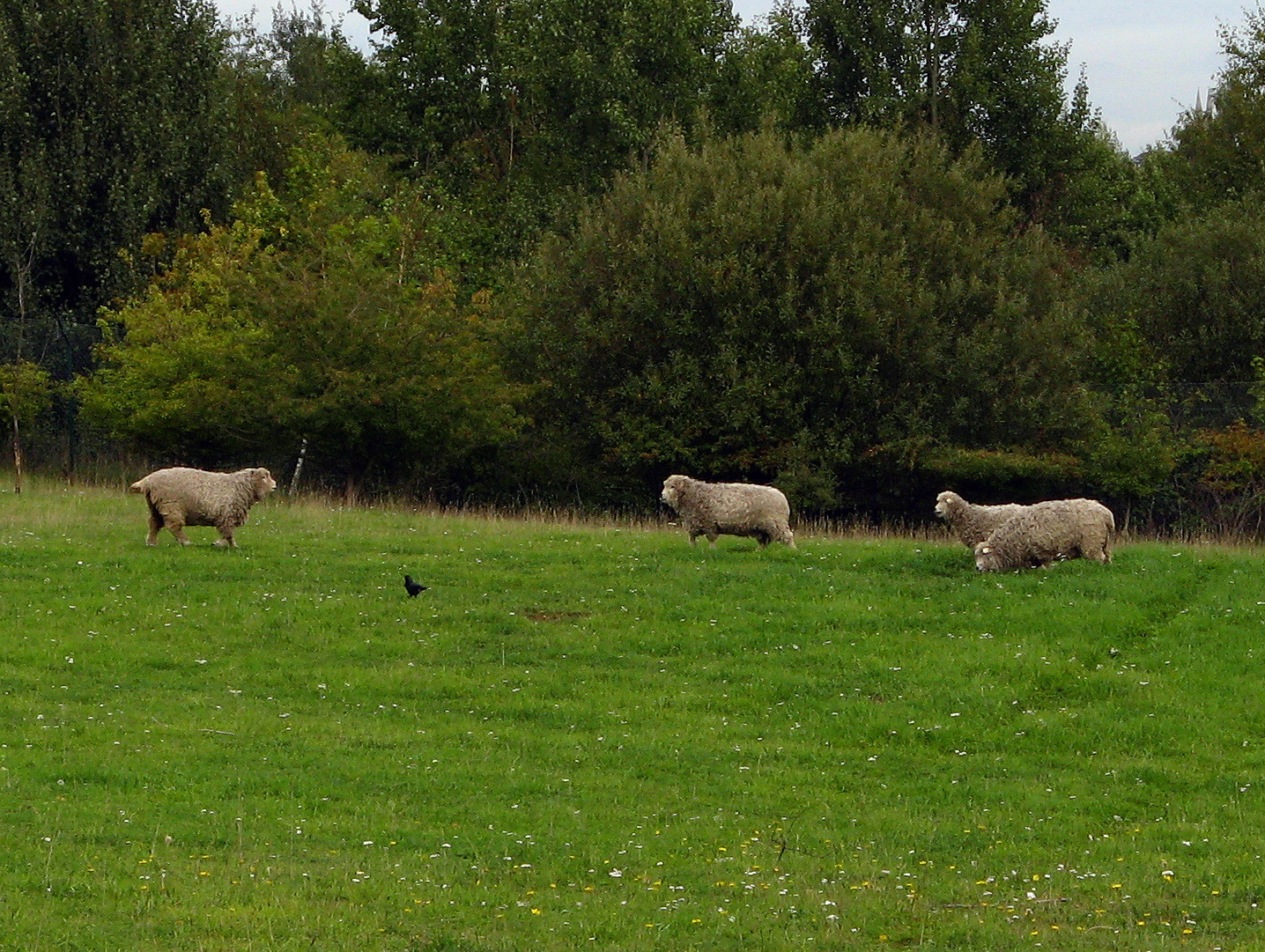In this outdoor photograph, the primary focus is on four fluffy, light gray sheep standing in a slightly sloped, green grassy field sprinkled with small white flowers and dandelions. The field is surrounded by lush trees and bushes, which appear darker green in the background and lighter green towards the front. The sky above the trees is a whitish blue, indicating a mostly cloudy day.

In the foreground, near the middle, a small black bird stands close to one of the sheep. On the left side of the image, one sheep faces to the right, with its tail visible as a small nub. To its right, near the center, a second sheep looks left, while slightly behind it, two more sheep also face left. Of the two at the back, one has its head down, grazing in the grass. Both of these sheep show only a partial view, with the fourth sheep slightly hidden behind the third.

The overall scene suggests a tranquil, open area where the sheep are either grazing or interacting with each other amidst the predominantly green, weed-filled grass, framed by a backdrop of mature, leafy trees.